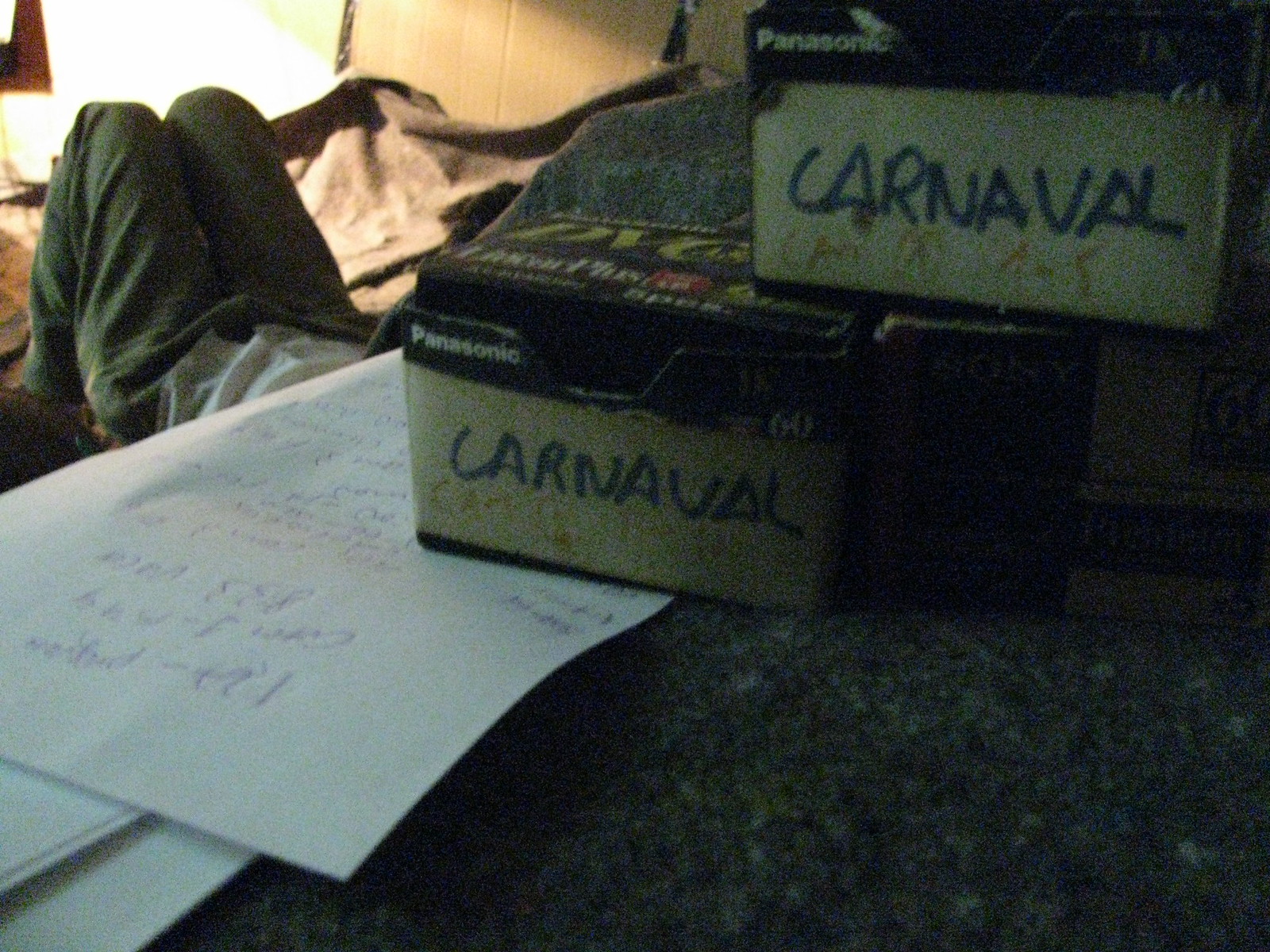This color photo depicts a close-up view of Panasonic VHS tape boxes arranged on a green countertop, each prominently labeled with "Carnival" in dark marker. Nestled among the Panasonic boxes is one Sony VHS tape box. To the left, there are white papers scattered on the counter, marked with blue ballpoint pen scribbles—possibly notes or calculations. In the background, a person is lying on a bed or couch, identifiable by their bent knees and feet flat on the surface, wearing a white t-shirt and dark pants. The scene includes a warm light emanating from the top left corner, which casts a brightening effect that contrasts with the darker, wood-paneled wall and the overall dimmer setting around the VHS boxes.